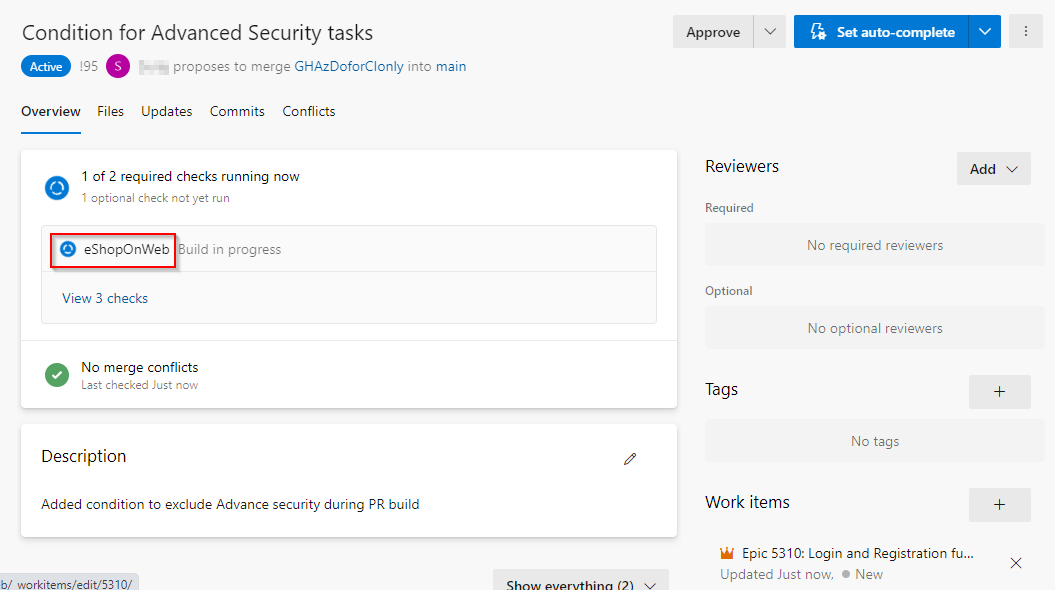This screenshot depicts a desktop interface with a predominantly light gray background. The top left corner features the title "Conditioned for Advanced Security Tasks" in black text. To the right of this title are two drop-down menus, one labeled "Approved" in gray and the other "Set to Auto-Complete" in blue, followed by a set of three vertical dots. Below the title is a blue "Active" button, and adjacent to it is a magenta circle, likely indicating some status or notification.

The screen then displays a project proposal titled "Proposes to Merge GHAZ GoFork Lonely into Main," with an "Overview" tab underlined in blue, denoting it is currently selected. Other tabs listed include Files, Updates, Commits, and Conflicts.

Below the tabs, there is a white box with one of the required checks currently running, identified by a blue logo. Nested within this section is a gray sub-box labeled "eShop on web," indicating that a build is in progress, along with the option to view three checks.

Further down, another white box contains a green logo with a white checkmark, signifying "No Merge Conflicts," with a note stating this check was completed "just now." A subsequent white box includes a description that reads "Added Condition to Exclude Advanced Security during PR Build." This box features a pencil icon for editing the text.

On the right side of the screen, there's a section for reviewers, featuring a drop-down "Add" menu with categories such as "Required" and "Optional," both currently indicating "No Required Reviewers" and "No Optional Reviewers." Below this section are options for adding tags and work items, both represented by a plus sign. Finally, there's an orange crown icon next to "Epic 5310 Login and Registration," marked as "Updated Just Now" with a status of "New," and an "X" icon to close it.